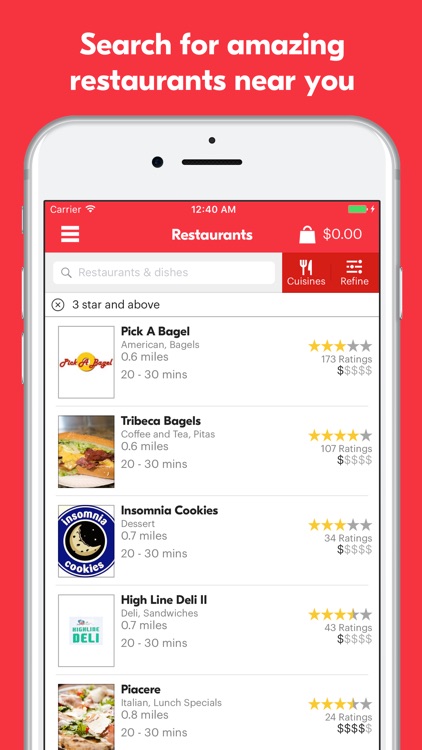The image showcases an advertisement for a restaurant app, depicted on a sleek gray phone. The background of the app screen is a vibrant red, with bold white text inviting users to "Search for amazing restaurants near you." The app prominently displays a tab for highly-rated options—specifically, restaurants rated three stars and above. Featured establishments include: "Pick A Bagel," "Tribeca Bagels," "Insomnia Cookies," "Highline Deli," and "Pi Sir." Each restaurant listing includes ratings and the variety of food available, providing users with essential details to make an informed dining choice. The ad captures the app's intuitive design and user-friendly interface, emphasizing its ease of use for finding quality dining options.